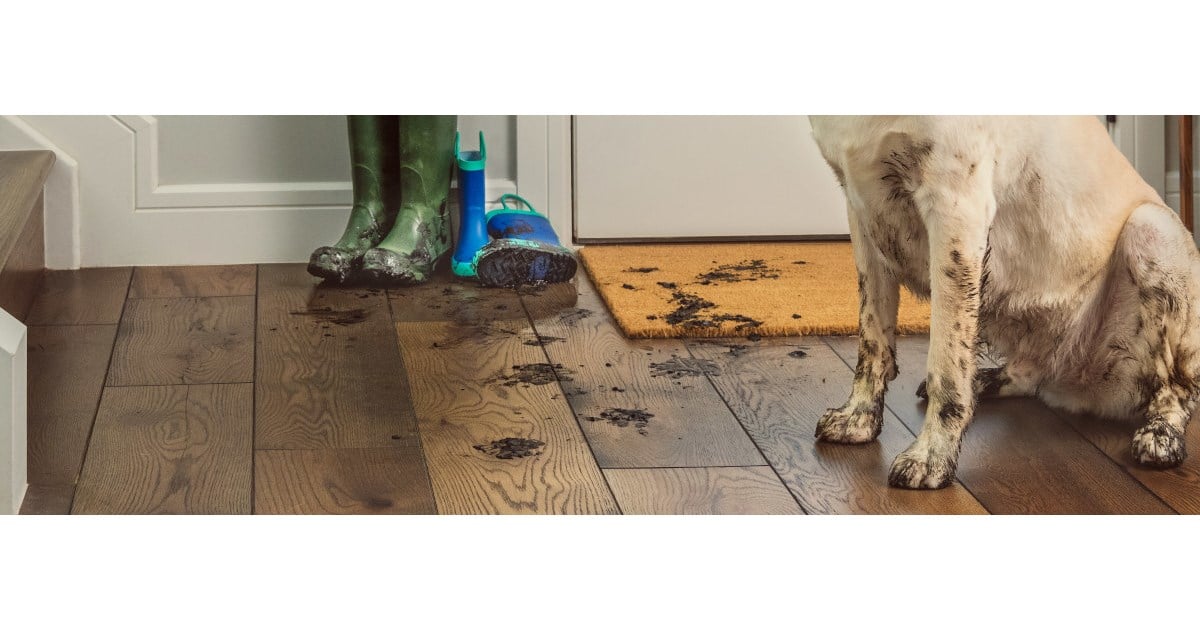This photograph captures a bustling and muddy entryway of a suburban home, immediately conveying a sense of recent outdoor activity. At the heart of the image is the bottom half of a medium-sized dog with light-colored fur, sitting on a dark hardwood floor. The dog's feet and tummy are caked with mud, leaving a trail of muddy paw prints scattered across the floor.

Prominently placed near the door, which is partially visible with its white bottom trim, are two pairs of muddy boots. One pair is an adult's green boots, standing upright, and the other is a child's pair, mainly blue with teal accents at the top and bottom. Directly in front of the door lies an orange doormat, also smeared with mud, further emphasizing the mess brought in from outside.

To the left of the scene, a glimpse of the bottom of a staircase can be seen. The wall is painted gray, but only a small section is visible above the white trim behind the boots. The overall scene vividly illustrates a common, albeit messy, slice of suburban life, emphasized by the muddy chaos at the entrance.